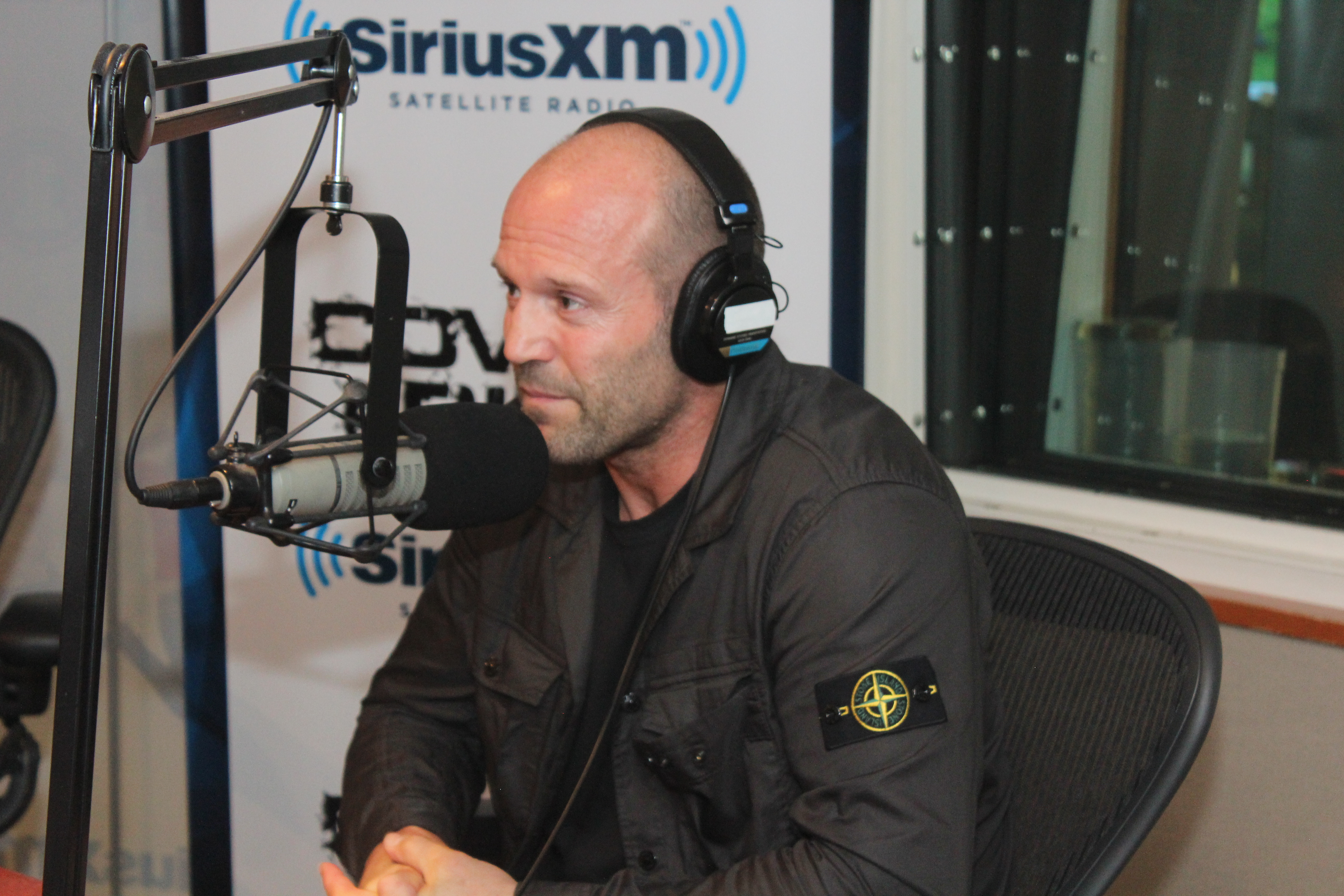The image depicts Jason Statham seated in a professional recording studio, evidently participating in a Sirius XM Satellite Radio talk show. Positioned in the middle of the frame, he sits on a chair in the lower right quadrant. In front of him is a microphone apparatus mounted on an adjustable arm, pointing toward his mouth, indicative of active engagement. He wears large headphones over his ears, with his hands folded, suggesting he is either speaking or intently listening. Statham is dressed in a black crew neck t-shirt and a jacket featuring a four-pointed star symbol encircled on its sleeve. Behind him, a window flanks his left side, while a wall bearing the text "Sirius XM Satellite Radio" occupies the background, emphasizing the setting. The color palette includes shades of black, beige to tan, green, white, light blue, dark blue, and burgundy red, adding depth and context to the professional studio environment.